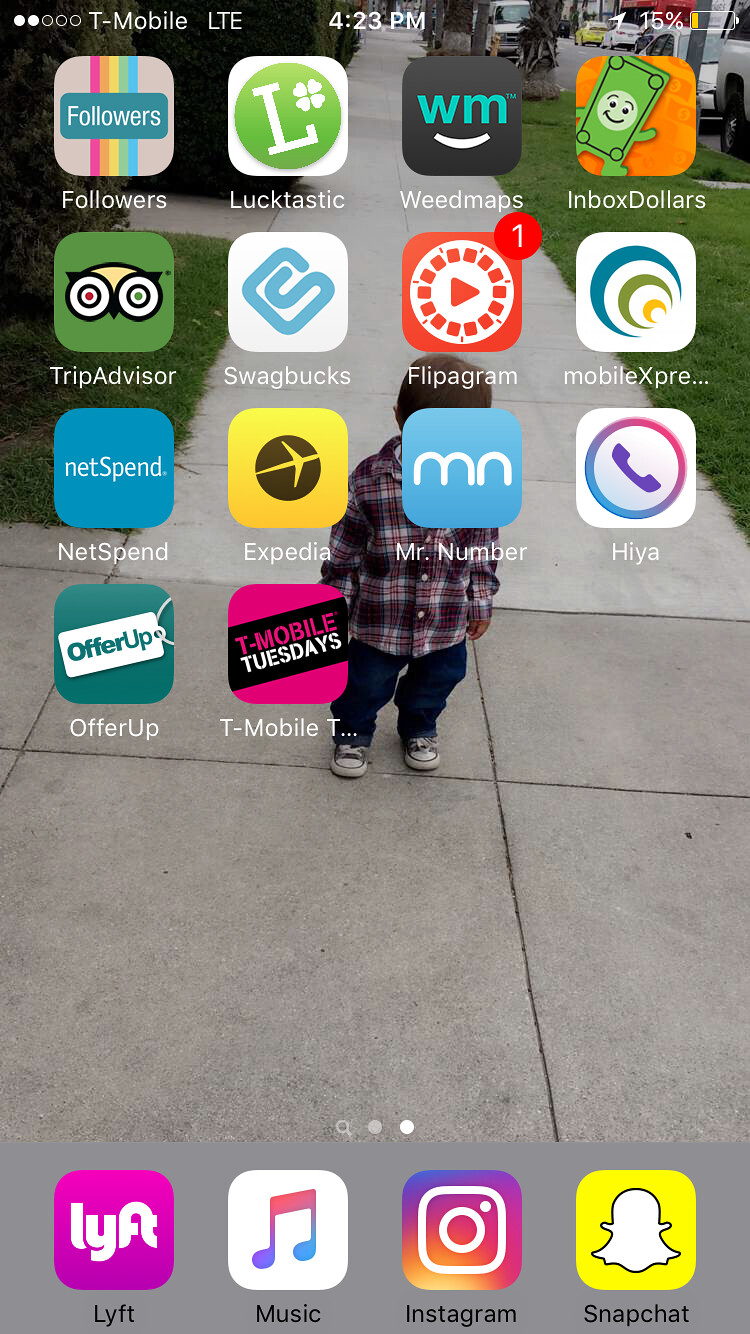A screenshot of a smartphone home screen showcases a custom wallpaper featuring a young boy, presumably the user's child. The child is dressed in black and white shoes with white laces, blue jeans, and a red, white, and blue plaid shirt. He has short brown hair and is standing on a gray sidewalk surrounded by green grass and shrubs, with cars parked along the side of the road.

At the top of the screen, the status bar indicates a T-Mobile network with LTE connection, two bars of signal strength, and the time displayed as 4:23 p.m. The location services icon is visible, and the battery is critically low at 15%.

The home screen contains several apps, organized in multiple rows. Visible app icons include Followers+, Looktastic, Weedmaps, InboxDollars, TripAdvisor, Swagbucks, Flipagram, MobileX, NetSpin, Expedia, Mr. Number, Hiya, OfferUp, and T-Mobile Tuesdays. The bottom tray features essential apps: Lyft, Music, Instagram, and Snapchat.